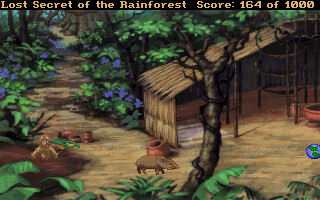This image is a low-resolution screenshot from a video game, which appears to be either a retro console game, a smartphone game, or possibly running on an emulator. Across the top of the image, there is a narrow black strip with yellow text displaying the title "Lost Secret of the Rainforest" followed by the player's score, "164 of 1000." The gameplay scene presents a basic but vividly depicted rainforest environment. The ground is primarily yellowish with patches of green, indicative of wear and erosion over time. In the middle-ground stands a rudimentary shelter made of straw and thatch, featuring a left wall and a sloping roof supported by sticks, giving it an open, temporary look.

In the background, dense green foliage can be seen, along with what appear to be blue-headed flowering plants adding color to the scene. Dominating the center of the frame is a wild hog or pig, contributing to the wilderness ambiance of the setting. The overall impression is of a small clearing or a makeshift dwelling in the heart of the rainforest, designed for survival and daily living amidst nature.